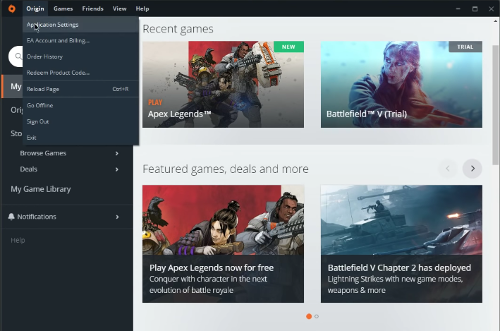Landing page screenshot for a video game website, showcasing various titles and offers. Four main panels dominate the right side:

1. **Top-left panel:**
   - **Game:** Apex Legends
   - **Text Details:**
     - "Play" (in orange)
     - "Apex Legends" (in white)
   - **Visuals:**
     - Two characters holding guns
     - White background with a red stripe
     - "New" label in a green rectangle with white text in the top-right corner

2. **Top-right panel:**
   - **Game:** Battlefield 5
   - **Visuals:**
     - A woman with a dirt-smudged face
     - Light blue background
     - "Trial" label in a black or gray rectangle with white text in the top-right corner

3. **Bottom-left panel:**
   - **Section Title:** Featured Games, Deals, and More
   - **Offer:** Play Apex Legends for free
   - **Visuals:**
     - Three characters wielding guns
     - Red background

4. **Bottom-right panel:**
   - **Game Add-on:** Battlefield 5 Chapter 2, Lightning Strikes
   - **Text Details:** 
     - New game modes, weapons, and more
   - **Visuals:**
     - Image of tanks

This layout effectively highlights the featured games and available offers, guiding users towards the latest releases and promotions on the site.